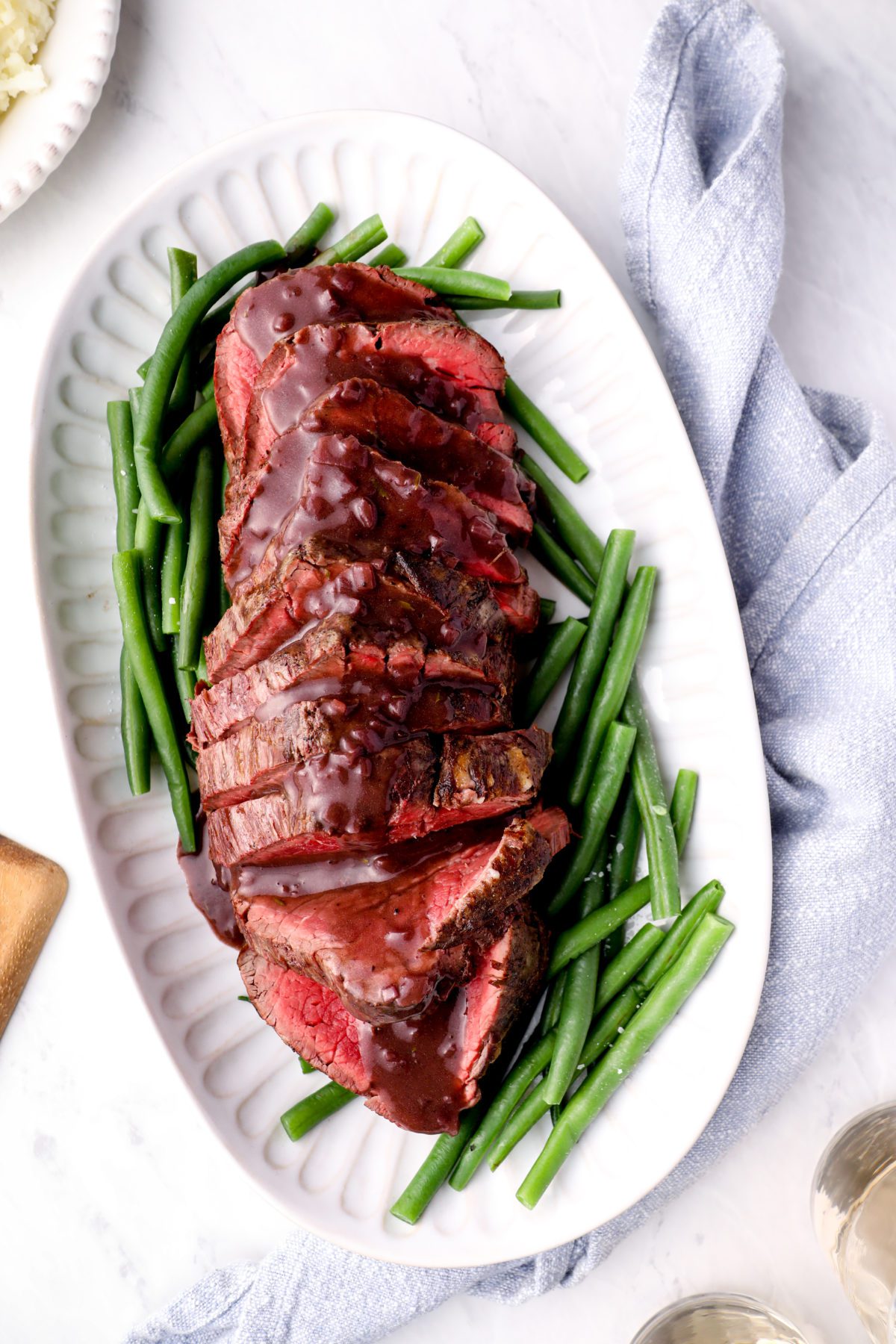The image features an overhead view of an oblong, white platter with an indented rim. On the platter sits a sliced roast of red meat, likely prime rib, which is brown on the outside and red and rare on the inside, radiating a somewhat bloody appearance. The meat is coated with a chunky, brownish-red gravy that might contain bits of vegetables. Encircling the roast are bright green beans, serving as a garnish. The platter rests on a white Carrara marble surface, partially overlapped by a folded light blue napkin on the right side. Accompanying the main dish, the upper left corner displays a similar white dish filled with what appears to be mashed potatoes, and the bottom right corner shows the rim of a glass, possibly alongside salt and pepper shakers. The bottom left hints at a brown item, which might be bread or another wooden item, enriching the scene with a variety of textures and colors.